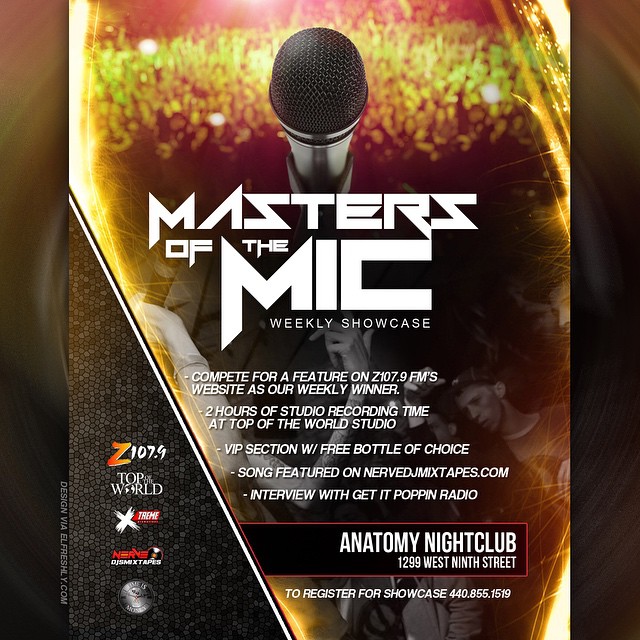The flyer is for an event at Anatomy Nightclub located at 1299 West 9th Street. The image features a black microphone with a silver handle positioned at the top, against a background that resembles yellow fireworks or golden sparkles. Below the microphone, in bold white sharp-edged letters, it reads "Masters of the Mic," followed by "Weekly Showcase" in smaller text. The details of the event are listed, encouraging participants to compete for a feature on Z107.9 FM's website as the weekly winner, two hours of studio recording time at Top of the World Studio, VIP section with a free bottle of choice, a song featured on NervedJMixTapes.com, and an interview with Get It Poppin' Radio. The background subtly shows an outline of a crowd and possibly a person holding a microphone. The flyer also includes logos for Z107.9, Top of the World, Xtreme, and two other indistinguishable logos, with the main colors being black, white, red, yellow, and gold. For registration, participants are directed to call 440-855-1519.